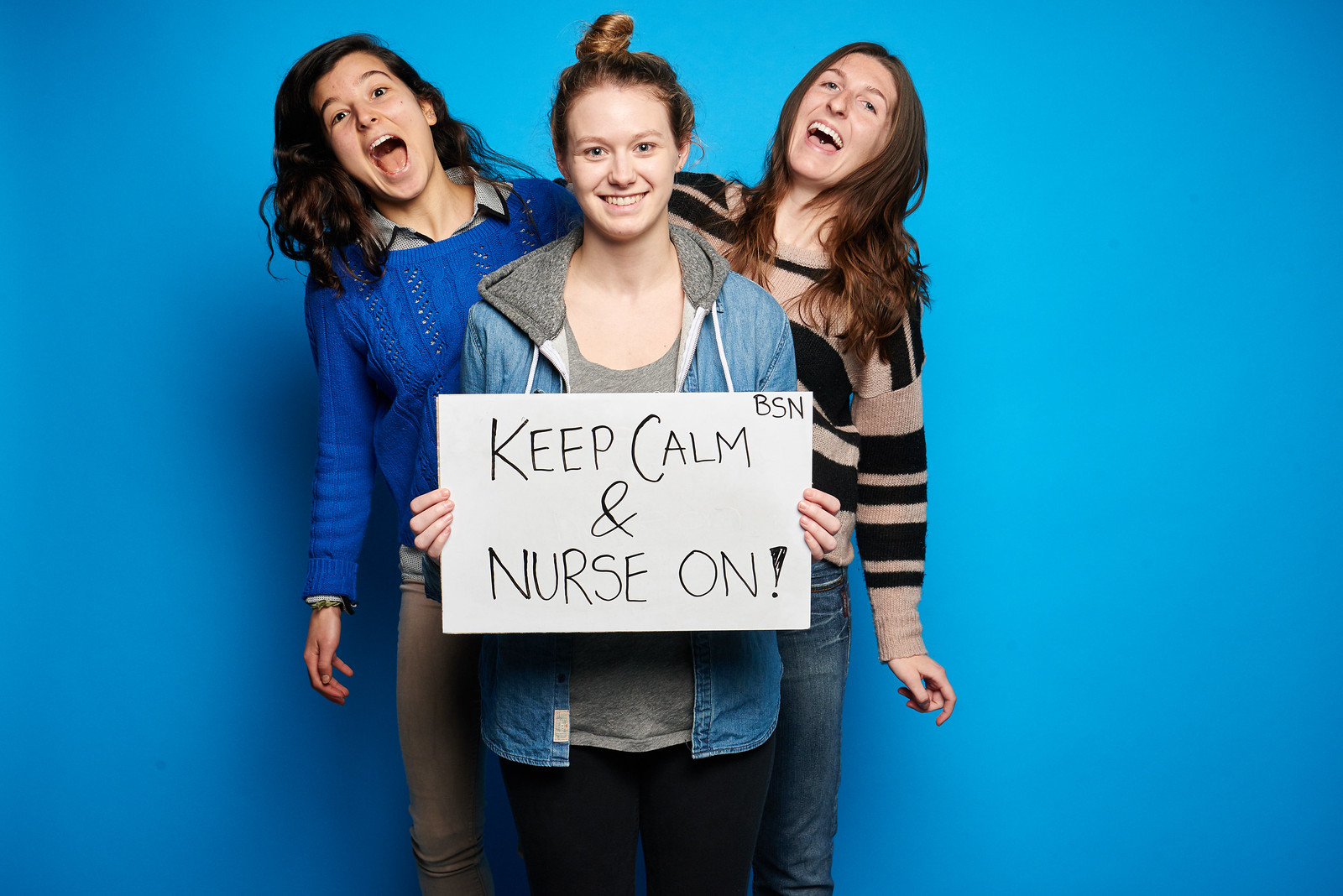The image features three women standing against a bright blue background, all of them smiling and laughing. In the center, a woman wearing a blue jean jacket over a gray hoodie and gray t-shirt holds a handmade white sign with the words "Keep Calm and Nurse On" written in black, along with "BSN" in the upper corner. She pairs her attire with black pants. To her left stands another woman, with long brown hair, dressed in a blue knitted jumper over a light blue collared shirt and brown pants. She is also posed with her mouth open, sharing a joyful expression. On the far right, the third woman sports a black and brown striped long-sleeved sweater paired with blue jeans, her mouth open in laughter and her long brown hair framing her face. The scene captures a moment of camaraderie and shared happiness among the three friends.